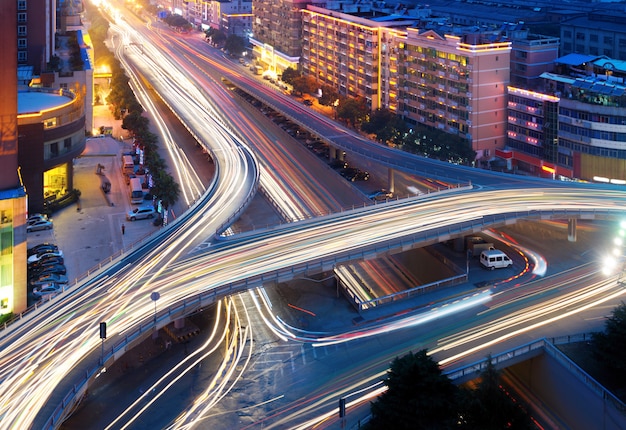The image appears to be an AI-generated, time-lapsed nighttime scene of a bustling freeway that cuts diagonally from the top left to the bottom right of the frame, ending in a loop and an overpass. The highway is adorned with bright white neon lines, creating a vibrant contrast against the dark surroundings. Flanking the freeway are an array of urban structures rendered in pastel hues. The left side showcases two tall buildings bracketing a shorter one with a large, brightly illuminated plate glass window. In the top left, a source of intense yellow light adds an enigmatic glow. On the right, high-rise apartment buildings stretch from the bottom edge up towards the center, each room illuminated in yellow, accentuating the evening setting. The entire scene lacks much greenery, save for a few scattered trees, and emphasizes the dense, intricate network of city infrastructure. The cars on the freeway are reduced to streaks of bright yellow and red light, highlighting the fast motion typical of a time-lapse capture, with some parked vehicles visible near the buildings. Overall, the photograph impressively captures a vivid urban landscape teeming with illuminated activity against the dark backdrop of night.